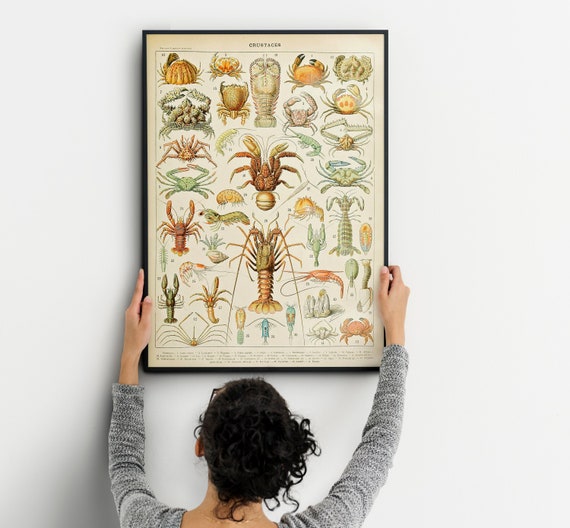The image depicts a woman with black hair tied in a ponytail, wearing glasses, hanging a framed piece of wall art on a white wall. The view is from the back, showing her head, arms, and shoulders as she carefully positions the artwork. The framed piece features detailed illustrations of various crustaceans, including crabs, lobsters, shrimp, and crawfish, arranged in an orderly fashion with around 20 different illustrations. The crustaceans are rendered in a range of muted colors, primarily greens, oranges, and yellows. The background of the artwork is a pale cream color, and the word "Crustacea" is prominently displayed at the top. The woman appears to be adjusting the frame to ensure it is level.